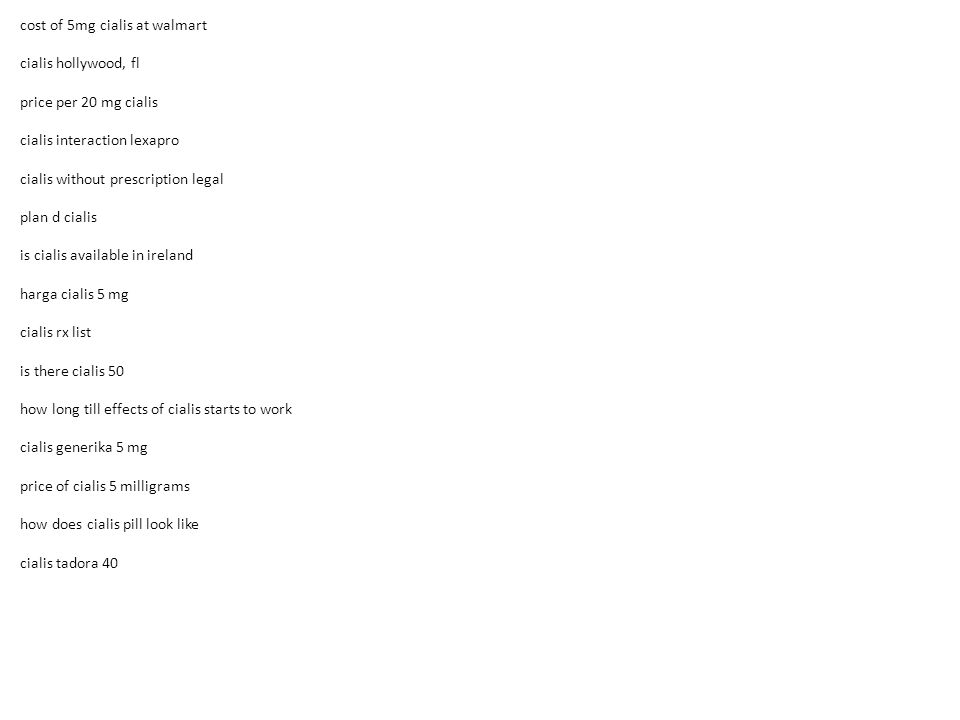Here is a more detailed and cleaned-up caption for the image:

---

**Category: Websites**

The image features a simplistic, text-based webpage with a stark white background. Positioned vertically along the left side of the screen is a concise, black-font list of search queries and topics related to Cialis. Each entry is in lowercase and directly pertains to information or queries about the medication. The list includes the following items:

- cost of 5mg Cialis at Walmart
- Cialis Hollywood Florida
- price per 20mg Cialis
- Cialis interaction with Lexapro
- Cialis without prescription legal
- Plan D Cialis
- is Cialis available in Ireland?
- Parga Cialis
- 5mg Cialis RX list
- is there Cialis 50?
- how long till effects of Cialis start to work?
- Cialis generica 5mg
- price of Cialis 5mg
- how does Cialis pill look like?
- Cialis Todora 40

The page does not contain any images, graphics, or additional text aside from this list, highlighting a focused search interest in various aspects of Cialis. The layout suggests the user's specific and immediate need for information regarding the drug.

---